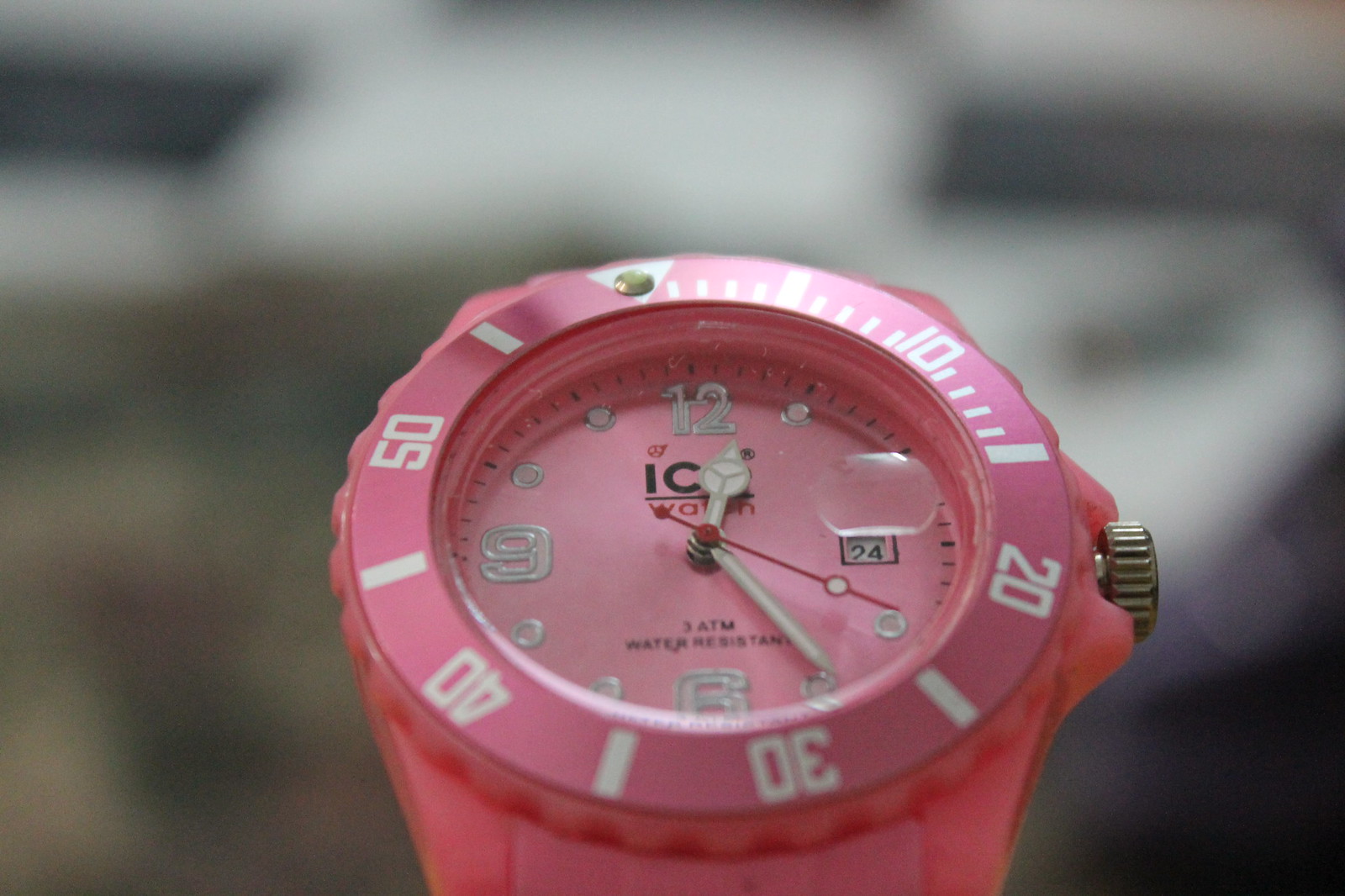A detailed close-up image showcasing a round, entirely pink watch captured from both a top and side view. The watch face is a vibrant pink, contrasting with white numerical markers adorning the interior. Each minute indicator is marked in black for precision. Surrounding the watch face, white lines and dashes delineate the outer rim, with larger numerals marking every ten minutes from 10 to 50. At the position where 60 would typically be, a distinctive white triangle marks the spot accompanied by a small, round metal piece. Beside the watch face, a dark-colored, ridged metal crown is visible, hinting at its function for winding or adjusting the time. The watch boasts a pink wristband, partially visible in the shot. The out-of-focus background features a blend of gray and white hues, ensuring the watch remains the image's focal point.